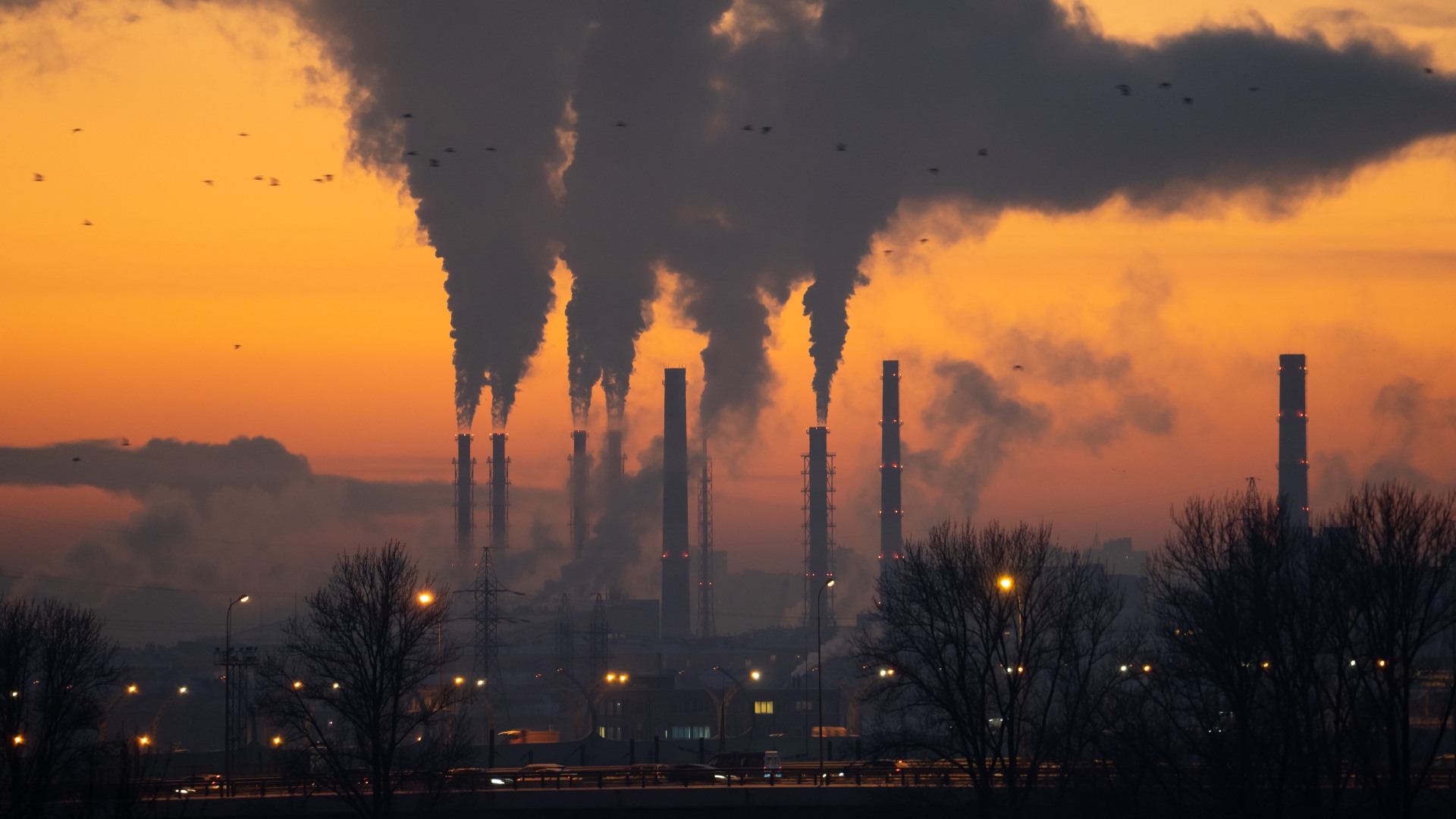A sprawling industrial landscape dominates the scene, punctuated by eight towering smokestacks that pierce an orange and yellow twilight sky. Dark gray and black smoke billows from six of these stacks, merging into a colossal cloud that blots out parts of the breathtaking sunrise. The factory complex below, possibly an oil plant, is illuminated with a mix of red, blue, yellow, and white lights, creating a stark contrast against the dark, looming structures. Surrounding the factory are leafless trees, which appear black against the dim light, and a highway bustling with cars, trucks, and a van. The highway, flanked by a black railing, stretches into the cityscape in the background, where more faint plumes of smoke can be seen, adding to the dense, industrial atmosphere.